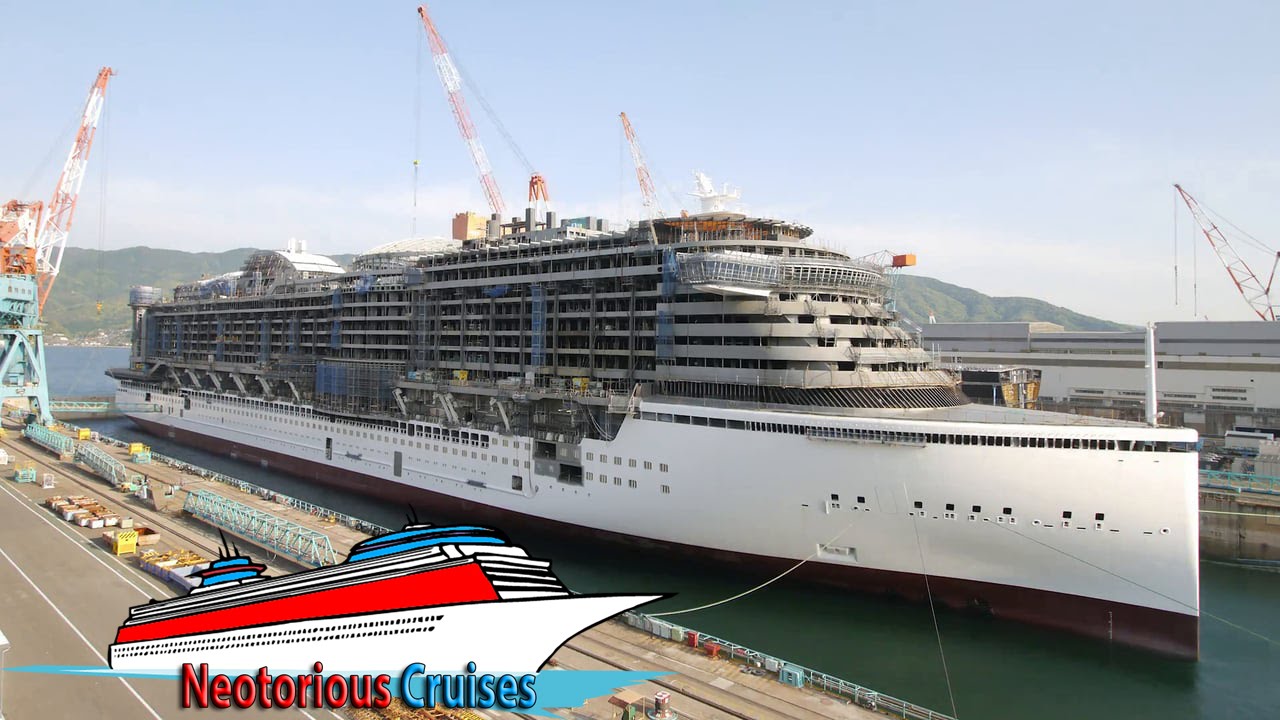This is a detailed photographic image of a massive, multi-story passenger cruise ship docked at a port during the daytime. The ship has a pristine white hull and an upper structure made of metal and glass. It is positioned behind several sloped elements, likely buildings. Prominent red and white cranes stand to both the left and right of the vessel, with another crane visible in the top right corner of the image. The clear, light blue sky serves as a backdrop, enhancing the scene.

In the foreground, there is a cement loading dock or parking area, with a path of medium blue water leading up to the ship. Additional water and distant hills can be seen in the background, emphasizing the outdoor setting. The ship's name, "Neotorious Cruises," is displayed in a mix of red, white, and light blue text at the bottom of the image, accompanied by a graphic of a white ship over a red background with blue and black chimneys. Various cranes occupy the area around the ship and though none are directly interacting with it, their presence suggests the ship might be undergoing some form of maintenance or loading activities.